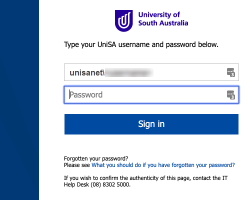The image shows a login window with a small, blurry interface against a white background. At the top, there is a logo resembling a shield, featuring a white design in the center, though the design details are unclear. To the right of the logo, the text "University of South Australia" is displayed in dark blue. Below this, in black text, instructions read: "Type your UniSA username and password below." There is a text field labeled "UniSANE," with the remaining portion blurred out, followed by a password input field. Beneath these fields, a dark blue rectangle with white text says "Sign In." Additional instructions below advise what to do if a password is forgotten: "Forgotten your password? Please read what you should do if you have forgotten your password." Further down, it states: "If you wish to confirm the authenticity of this page, contact the IT Help Desk at 06-8302-5000." A dark blue vertical bar extends along the left side of the window from top to bottom.